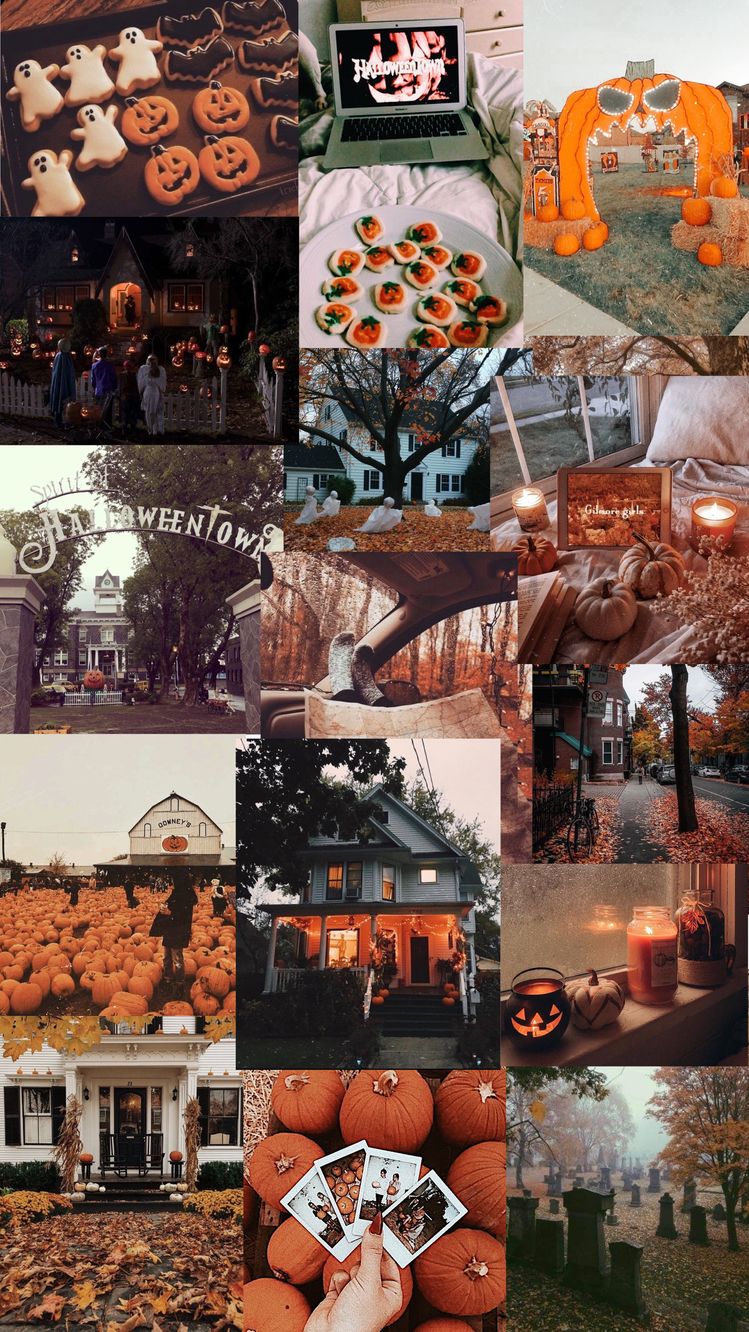This Halloween-themed collage depicts a variety of festive and spooky scenes, starting from the top left:

1. A delightful assortment of Halloween cookies shaped like ghosts, pumpkins, and bats.
2. A cozy image of someone lounging on their bed, munching on cookies while watching a movie featuring a pumpkin on their laptop screen.
3. A vibrant fair with a whimsical entrance designed to resemble a giant pumpkin's mouth.
4. Children standing outside a house adorned with numerous glowing jack-o'-lanterns.
5. A picturesque white house with a tree in front, surrounded by small, eerie ghost decorations on the ground.
6. An inviting, neatly made bed accented with pumpkins and softly glowing candles.
7. A relaxing scene of someone resting their feet up in a car.
8. A spooky gate labeled "Halloweentown," evoking a sense of mystery and holiday spirit.
9. A vast pumpkin patch with a quaint house situated in the background.
10. Another charming white house, this time highlighted in an orange glow, capturing the essence of Halloween decor.
11. A window ledge adorned with pumpkins and candles, creating a warm and festive vibe.
12. Yet another white house, complemented by a scattering of colorful autumn leaves in the foreground.
13. A vibrant display of pumpkins, notably one with faces carved into them.
14. A somber yet intriguing cemetery scene characterized by various tombstones.

The entire collage is unified by a palette of warm oranges, grays, and browns, encapsulating the essence of Halloween.